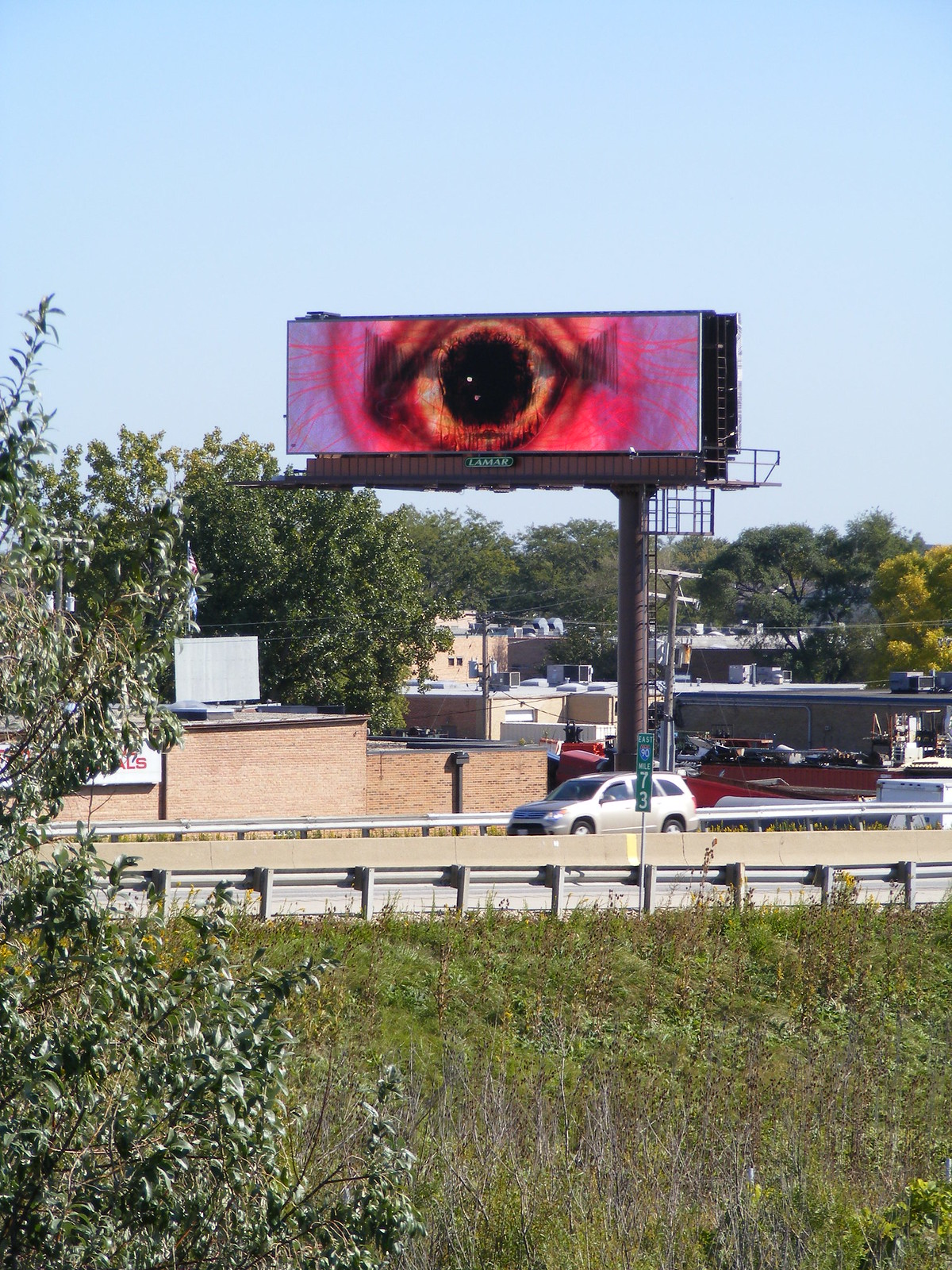This outdoor photograph captures a dynamic roadside scene from the other side of a median. In the foreground, there's a stretch of overgrown wild grass, mingling shades of light and dark green with patches of brown. On the left, taller bushes and trees with green leaves add depth. A silver or gray guardrail lines the gray concrete road, with a silver SUV driving along it. Across the road, a dominant billboard stands tall on a large black or brown cylindrical pole, featuring a vivid, AI-generated eye. The eye has a dark black pupil, transitioning through shades of yellow, pink, and hot pink to a striking purple on the outer edges, creating a surreal impression. Behind the bold billboard, a vibrant blue sky frames a background of trees and a mix of gray and tan buildings, while cars populate a parking lot. The detailed scene is completed by a concrete divider with a yellow stripe and a green and white mile marker labeled '73', contributing to the intricate roadside tapestry.